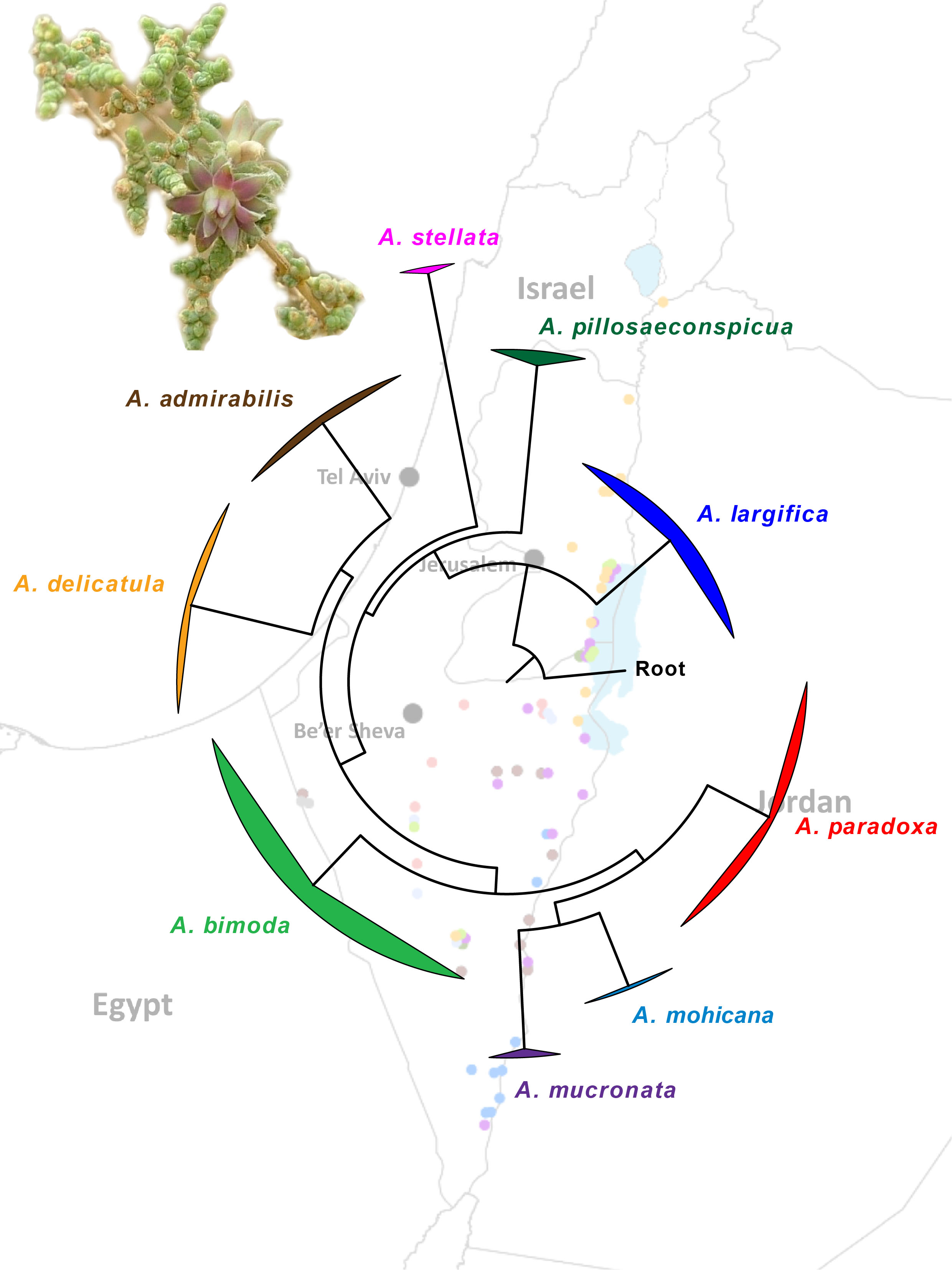This detailed image presents a map of Israel and surrounding countries, displaying geopolitical boundaries with labeled cities such as Tel Aviv, Jerusalem, and Beersheba. The map is situated on a white background with faint gray lines outlining Egypt to the southwest and Jordan to the east. Two pale blue bodies of water, likely the Mediterranean Sea to the west and the Dead Sea in the south, are also depicted. An intricate overlay features an enlarged, circular diagram at the center, marked by radiating lines that suggest a graphical representation of data. These lines are adorned with colored umbrellas, each tagged with a capital "A" and various scientific plant names like Paradoxa, Mohicana, Makronada, Bimoda, Delicatulia, Admirabilis, Stellate, Pilosaiconspicua, and Largifica. This diagram seems to correspond with a photo of a green, cream, and pink plant displayed in the upper left corner of the image, hinting at the distribution or characteristics of different plant species across the map.